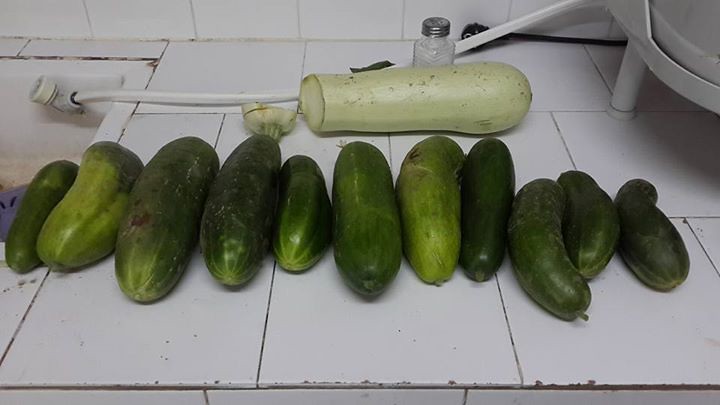In this color photograph displayed in landscape format, we see a white-tiled countertop, characterized by dark grout lines that highlight its aged appearance with dings but overall cleanliness. Arranged vertically on this countertop are eleven garden-fresh cucumbers, showcasing a variety of shapes and sizes, from dark green to a lighter, almost white cucumber. This pale cucumber has its top sliced off, which is conspicuously laid on its side in the background. The cucumbers, some with brown splotches indicating natural imperfections, are the focal point, lined up in order.

To the left side of the image, a portion of a white sink is visible, connected to a white-legged piece of equipment with a hose extending into the sink. Among the items on the countertop is a clear crystal salt shaker with a silver top. The scene is set against a backdrop of white porcelain tiles, suggesting a kitchen environment.